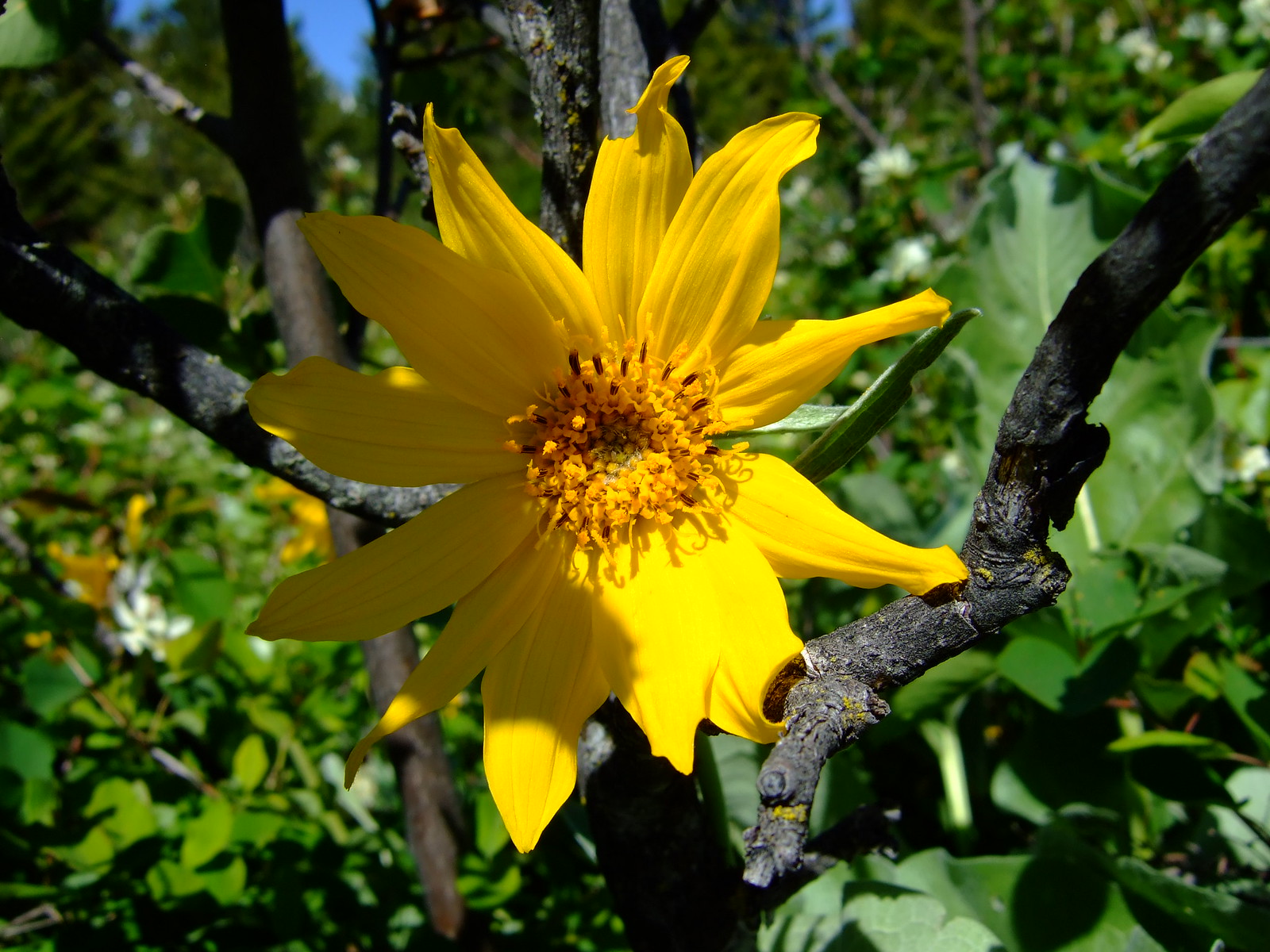The image showcases a vibrant yellow sunflower in full bloom, with exactly twelve petals radiating from its center. The core of the flower is a deeper, darker yellow-orangish hue, likely the focal point for pollination. This sunflower emerges prominently from among several bare branches, suggesting a stark contrast between its bright vitality and the sparse surroundings. The backdrop reveals lush green foliage, indicating a forest or garden setting, with more hints of sunflowers dispersed throughout. The sun shines brightly, casting light on one side of the flower and illuminating a crystal-clear blue sky. The overall scene exudes a sense of springtime, capturing the essence of natural beauty on a sunny day.